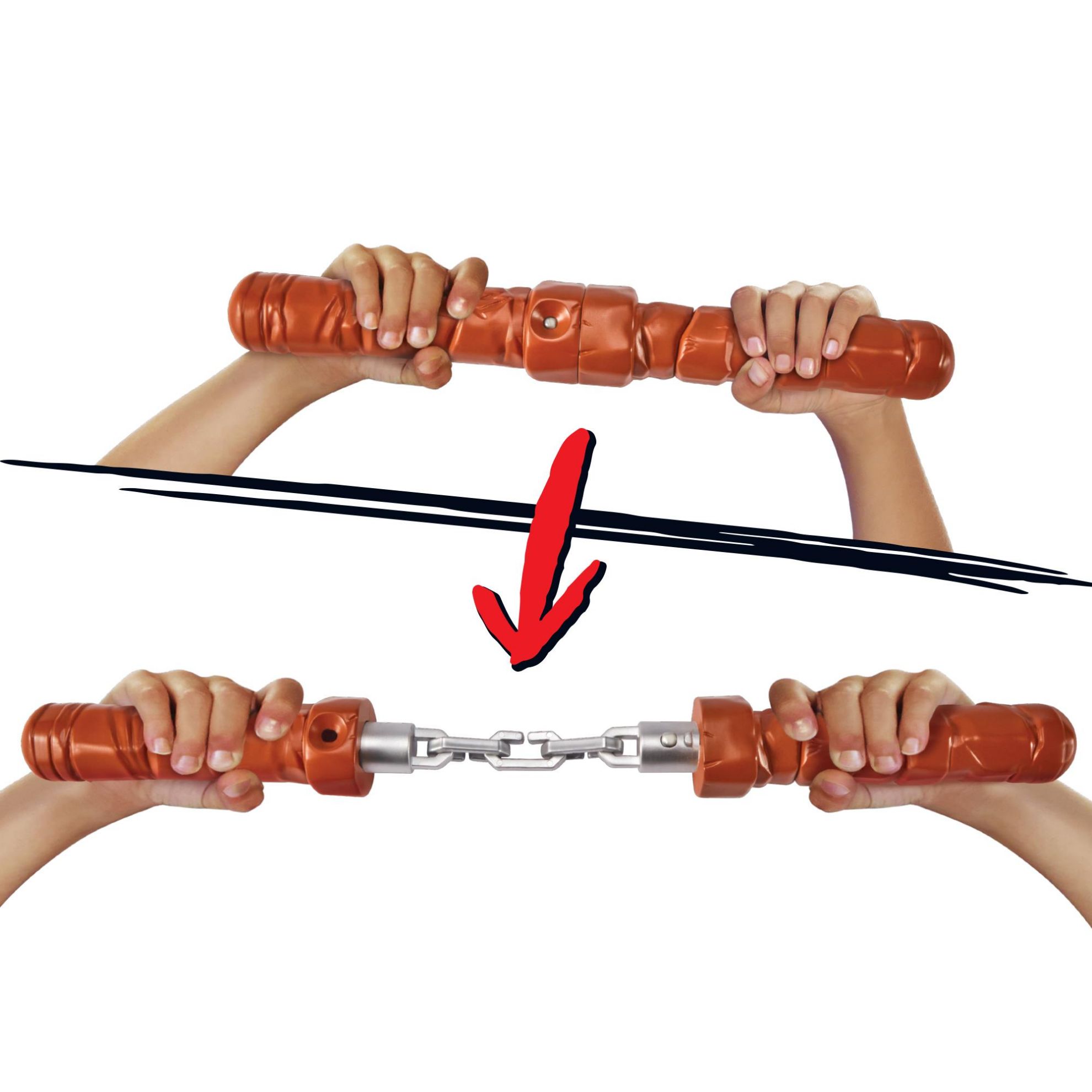This composite image displays a pair of toy nunchucks with prominent orange handles. The image is divided into two sections: the top section shows two hands holding the nunchucks closed together, while a red arrow points to the bottom section. In the bottom section, the same hands have pulled the nunchucks apart, revealing a silver chain linking the two handles. The chain appears to be made of plastic and features a small gap, suggesting it can be detached. Additionally, a black line separates the two sections of this before-and-after demonstration, underscoring the transformation from the nunchucks being closed to opened. The nunchucks themselves, short and thick with visible buttons on the handles, might include features such as flashlights or batteries.